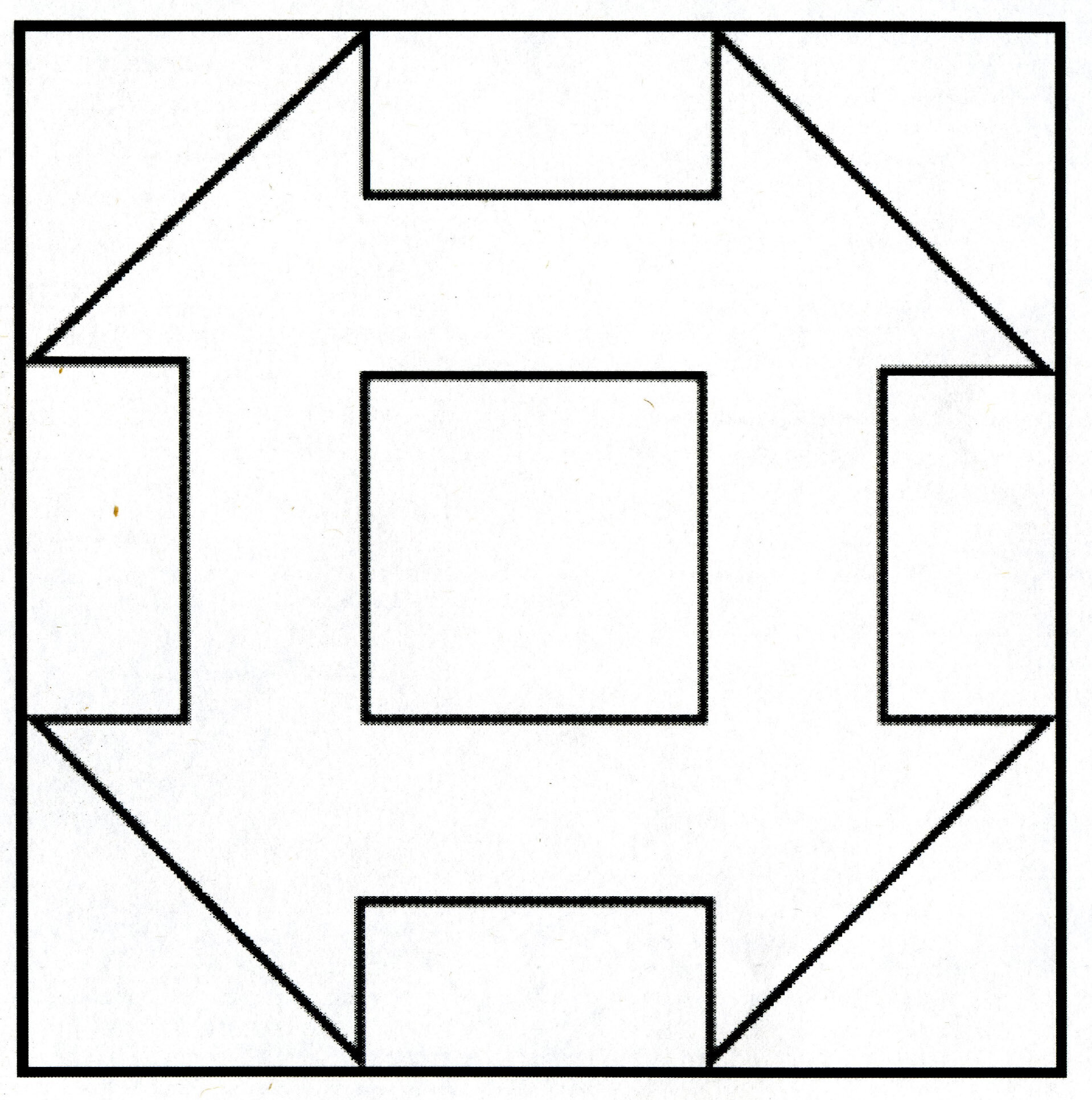The image features a simple yet perplexing geometric design composed of black lines on a white background. The overall shape is a square, within which lies a smaller central square that occupies about one-eighth of the total area. From each side of this central square extend four rectangular regions, each sharing the same width but only half the height of the central square, aligned at the top, bottom, left, and right. Additionally, each corner of the larger square contains a diagonal black line, transforming these corners into black triangles. The result is a symmetrical and repetitive pattern where the central square is flanked by rectangles, and the corners are sectioned off as triangles. This intricate arrangement creates a unique, symmetrical design that resembles a series of directional arrows or perhaps even parts of a lantern when viewed from different angles. Despite its simplicity, the pattern is detailed and intriguing, with its precise geometric form and contrasting black-and-white color scheme.